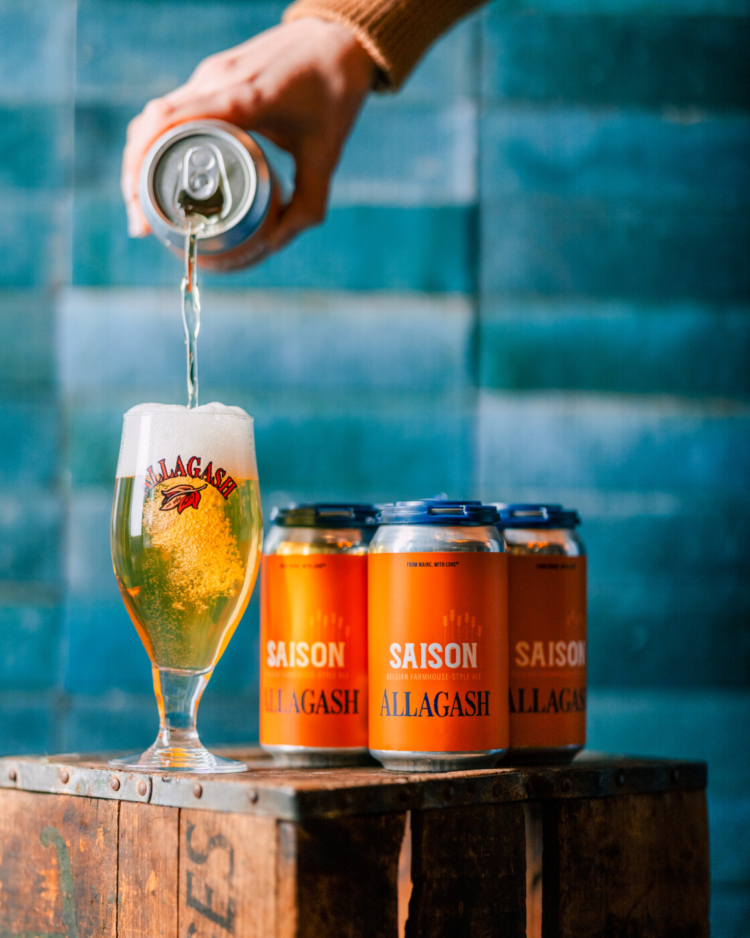A person pours a nearly overflowing glass of yellow beer from an orange-labeled can marked "Saison Allagash" in a detailed photograph. The foreground features a rustic wooden crate topped with two additional crates, one arranged horizontally and one vertically. Adjacent to these crates sits a transparent beer glass adorned with red "Allagash" lettering. Surrounding the glass are four orange cans of "Saison Allagash" beer. A hand, emerging from the upper part of the image, is captured mid-pour as the frothy beer flows into the glass. The scene unfurls against a weathered blue wall composed of individually laid panels, their paint faded and weather-worn, adding a textured, slightly blurry backdrop.